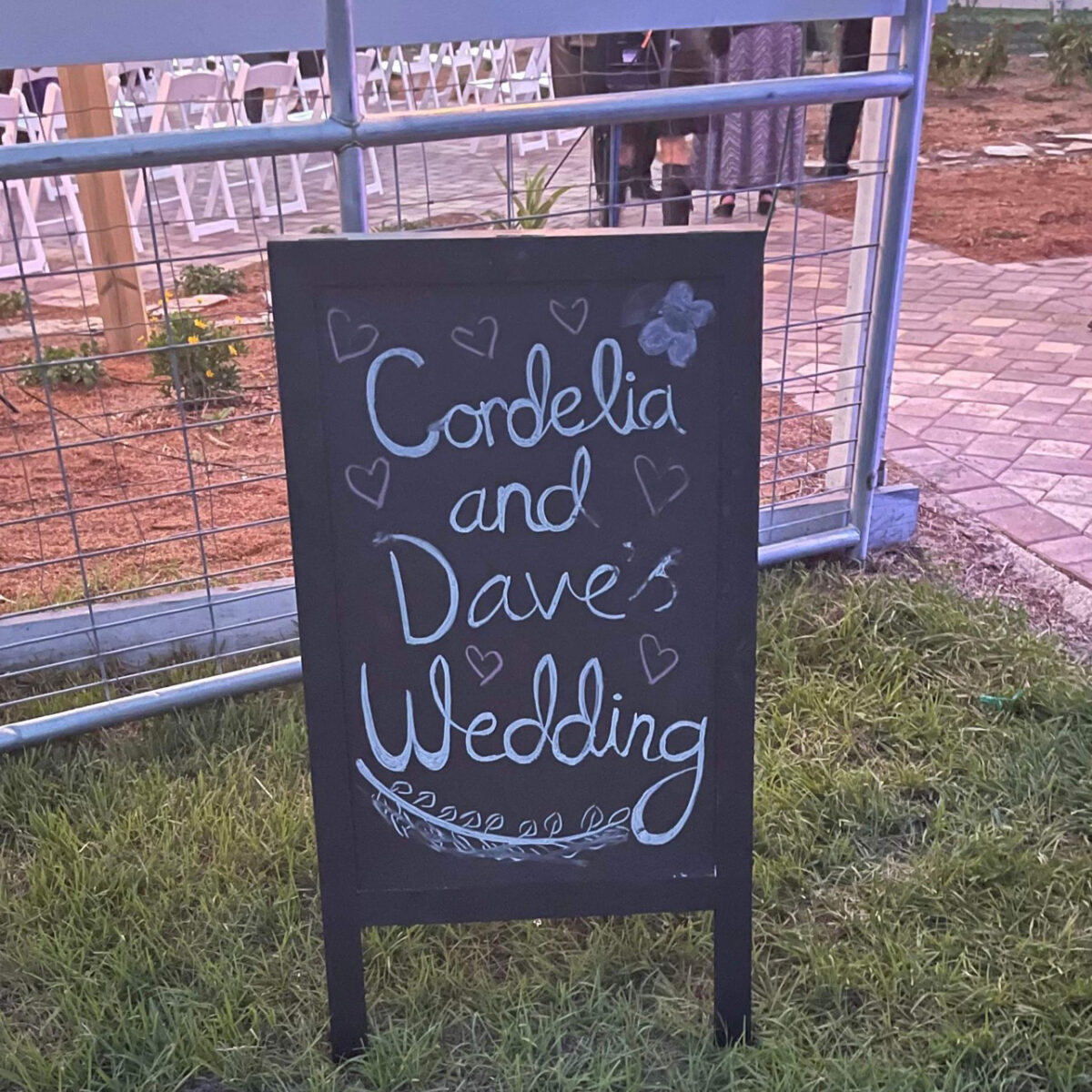This photograph captures a charming wedding setting centered around an elegantly decorated black sandwich board. The board, standing on a patch of lush green grass, reads "Cordelia and Dave's Wedding" in light blue chalk, adorned with artistic details such as hearts, a butterfly, and a vine-like sketch of leaves. Surrounding the sign is an intricate background that includes a large blue-gray fence and muddy, sandy grounds dotted with newly planted greenery. White folding chairs arranged for the ceremony are visible in the top left, while the legs of attendees, one wearing a kilt and another in a long blue skirt, add life to the scene. To the right, a beige-brown stone tile pathway borders the grass, leading into a space with more mud and footpaths, completing this picturesque wedding setup.